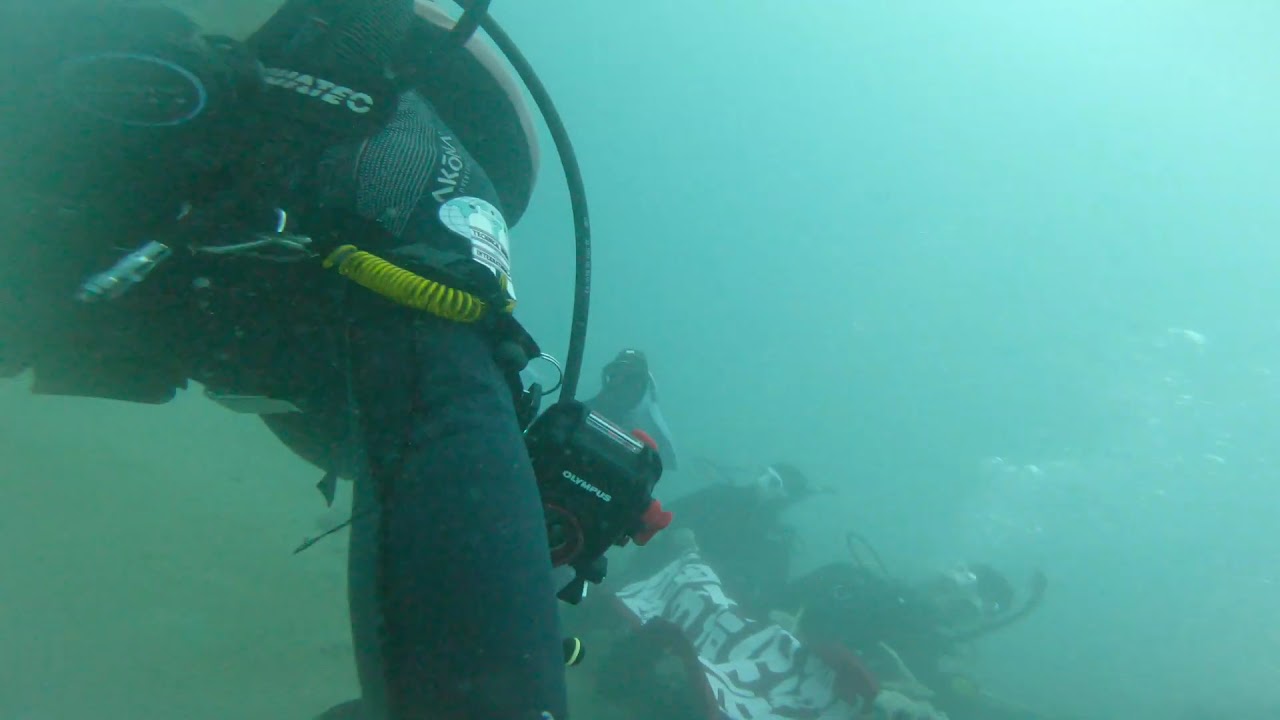The image captures an underwater scene where visibility is limited due to murky, greenish-blue water. Situated in the ocean, the photo appears to be taken in the middle of the day. On the left side of the image, a diver, possibly the one holding the camera, can be seen in a black and gray skin suit with a regulator visible. The diver seems to be taking a selfie with three other divers who are positioned towards the bottom of the image. These three divers, also in black diving suits, are holding a fabric sign featuring red and white lettering that looks like it is written in a Middle Eastern language. The sign has a zebra-like pattern in some spots. Additional colors present in the image include light blue, tan, silver, and yellow. The overall composition has the divers mainly located in the top left and bottom areas, with the rest of the image being relatively empty.